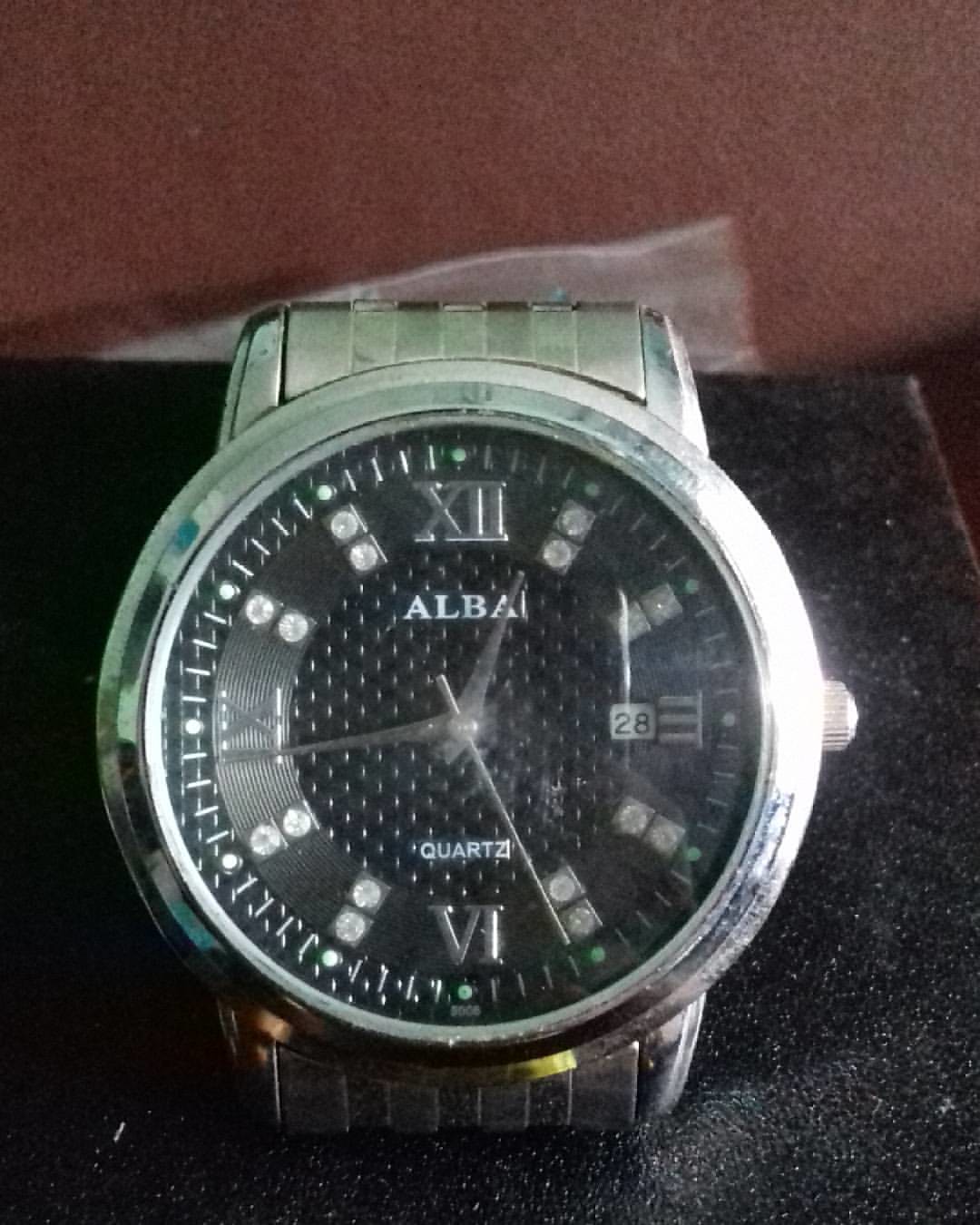This detailed photograph captures a close-up of a silver wristwatch, specifically an Alba quartz model, positioned on the corner of a black surface. The watch is set against a backdrop that includes a reddish-brown wall, with a piece of white fabric visible between the black surface and the wall. The wristwatch is notably large and designed for men, characterized by its hefty and bulky build. 

The band and faceplate of the watch are silver, while the watch face itself is black with a textured, dotted pattern. The inner ring of the watch face houses Roman numerals at the 12, 3, 6, and 9 o’clock positions, with the remaining hour markers represented by what appear to be small diamonds. The hands of the watch, which include hour, minute, and second indicators, are also silver. A date window is visible next to the 3 o'clock position, currently displaying the 28th. Additionally, there is some noticeable wear around the outer silver edge, suggesting the watch is not brand new. The time displayed on the watch is 12:44.

The entire composition is further complemented by subtle details, such as pieces of carpet and possibly plastic visible in the background, adding context to the placement of the watch within a seemingly domestic setting. The text "Alba quartz" is prominently displayed on the watch face in white, emphasizing its brand and type.